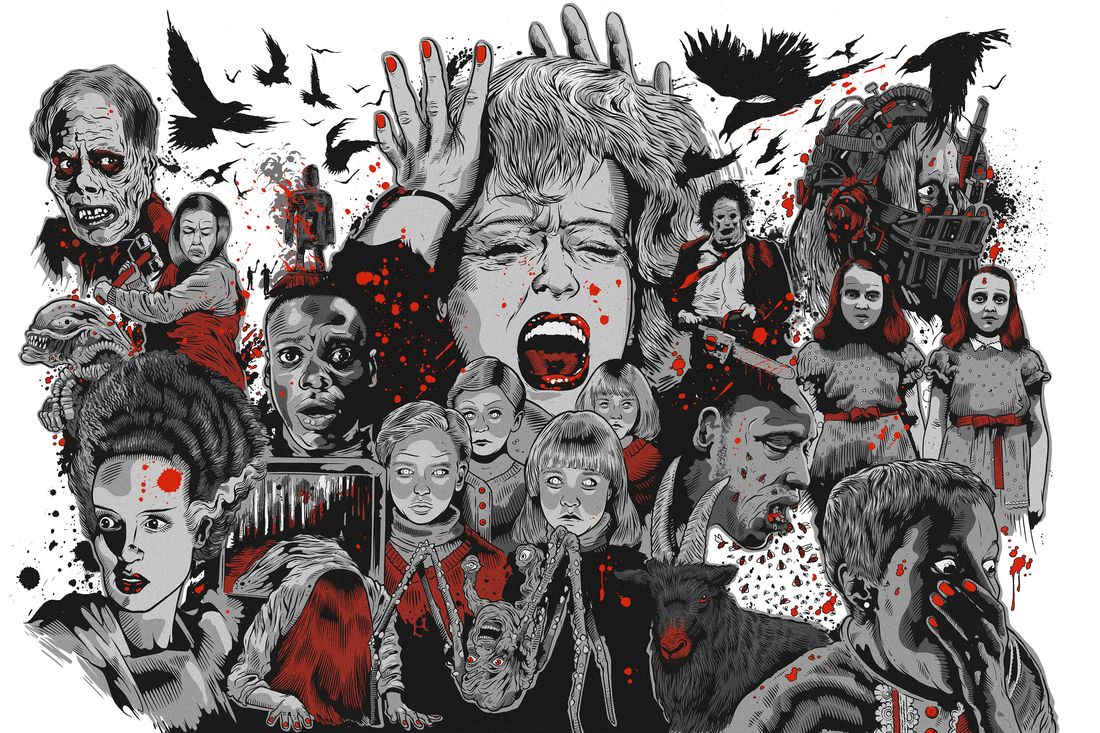The artwork is a highly detailed horror-themed piece, predominantly in black, white, and red, that seems to be a collage of various thriller and horror movie references. At the center of the image, a large, fear-stricken woman with short hair and blood splattered across her face dominates the scene, with her hands on the sides of her head, showcasing missing and strange-looking thumbs. Surrounding her are multiple terrifying elements: in the top left corner is a zombie-like man, while on the top right is a disturbing saw scene. Crows ominously fly around, especially near the woman's head, heightening the sense of dread. 

On the right side, two twin girls, reminiscent of characters from classic horror films, gaze eerily, and below them, a young boy with red fingernails and blood on his face stands out. To the left, fearful women with red hair scream in terror. The bottom of the piece features unsettling imagery including a horned animal with a bloodied mouth and a monstrous figure with eyes and tentacles. Throughout the image, various horror figures like a masked man in the top right, possibly resembling Freddy or Michael Myers wielding a machete, and blood-splattered children with zombie-like eyes contribute to the chaotic yet captivating scene. Cultural references abound in this busy, fear-inducing masterpiece, from chainsaws to hammers, creating a nightmarish panorama of horror.